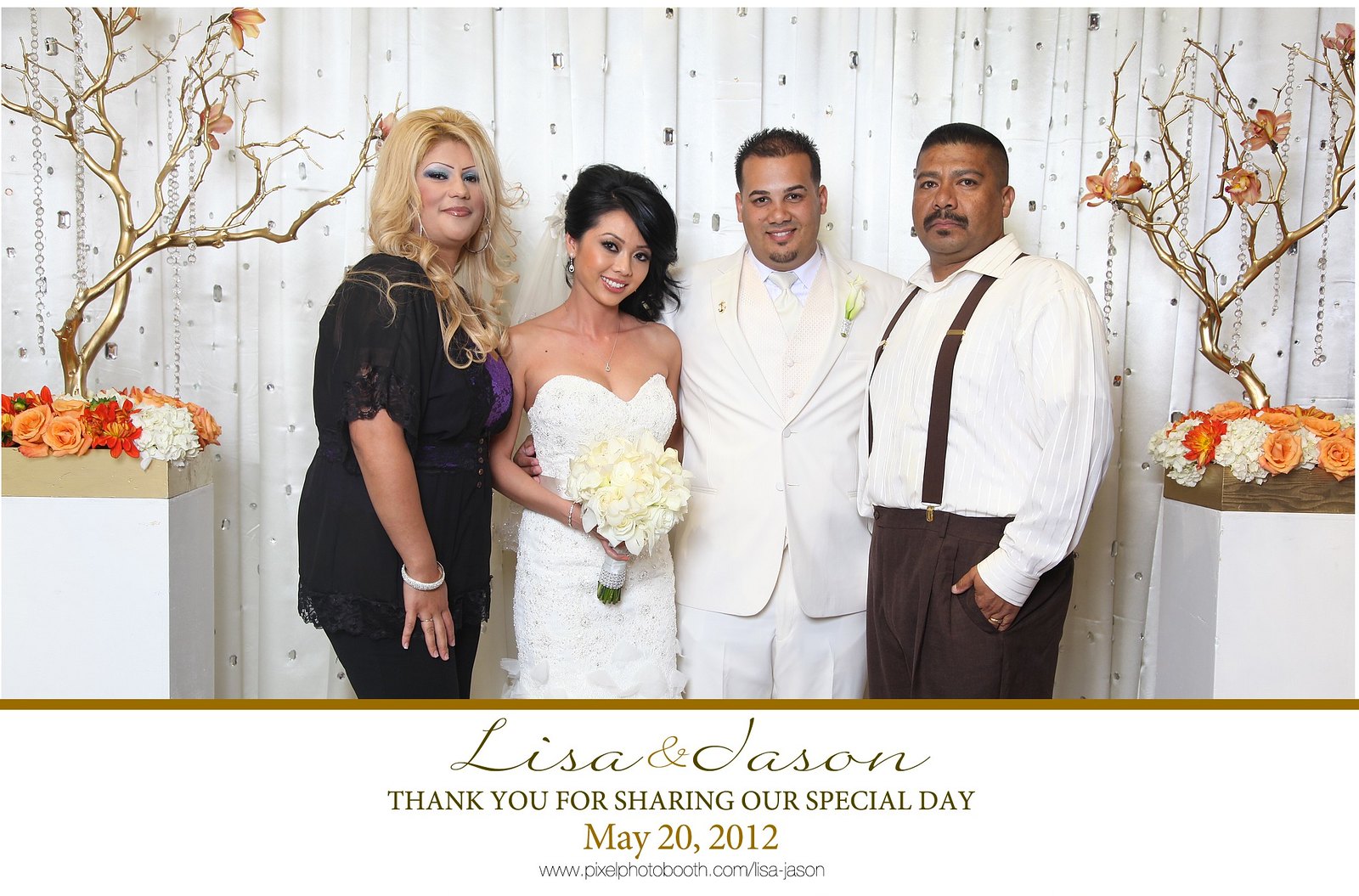The image depicts a wedding photo featuring four individuals against a white backdrop with silver accents. In the center stand the bride and groom. The bride, a medium-skinned young woman, possibly Italian and likely in her twenties, wears a form-fitting, strapless white wedding dress and holds a white bouquet of flowers. The groom beside her has short, spiky black hair and a chin beard, dressed in an off-white suit. Flanking the couple are another man and woman. To the groom's right is a man of apparent Mexican heritage wearing a white dress shirt, brown pants, and brown suspenders. To the bride's left is a taller Caucasian woman with blonde hair, wearing a black dress and blue eyeshadow, with a hint of a purple shirt underneath. The background is adorned with red, orange, and white flowers, positioned at the base of gold, leafless trees, adding an elegant touch. At the bottom of the image, text reads, "Lisa and Jason, thank you for sharing our special day, May 20th, 2012," along with the URL "www.pixelfotobooth.com/Lisa-Jason."